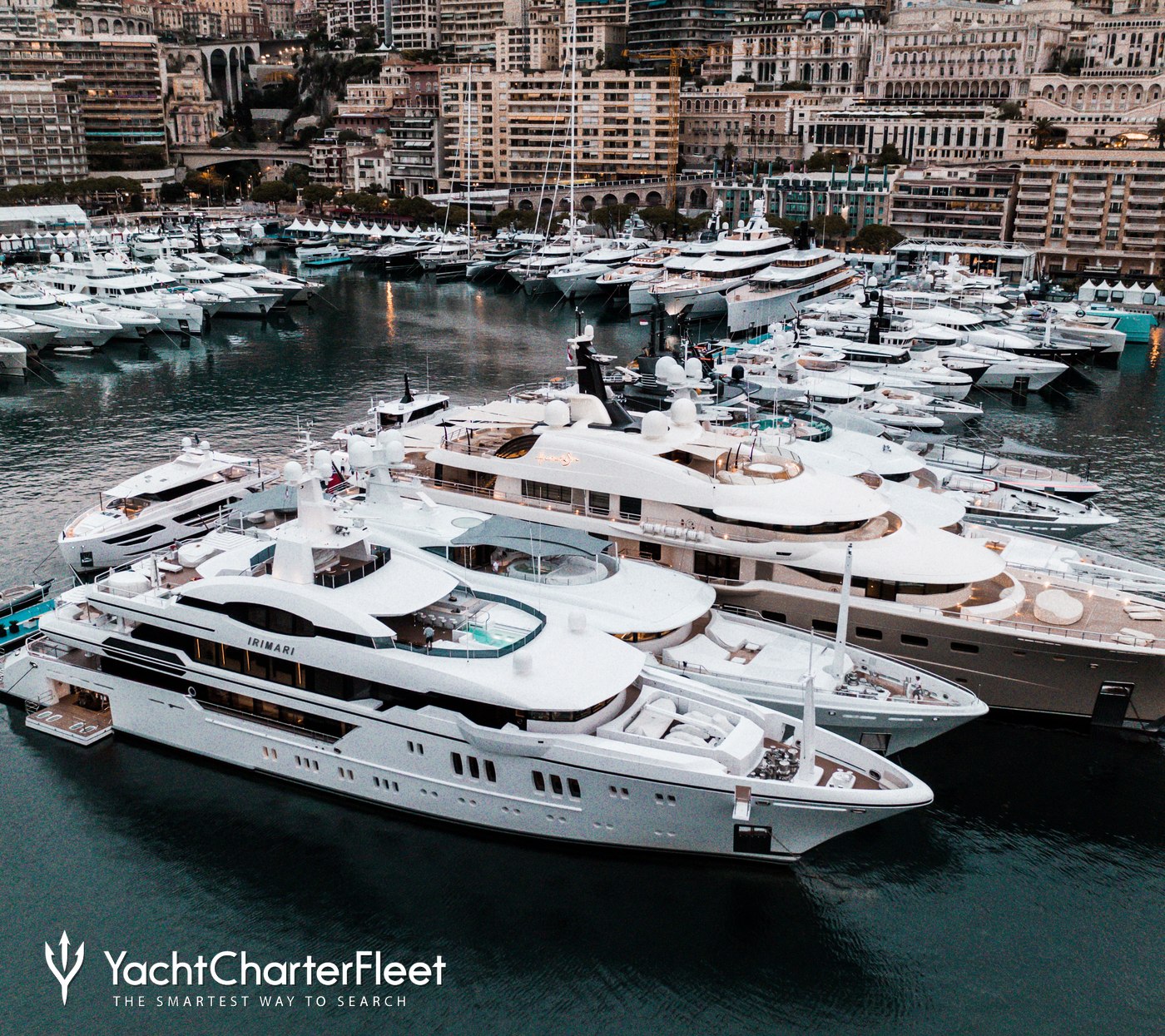The image depicts a bustling marina, featuring an array of dazzling yachts docked along a pier. In the bottom left-hand corner, written in white font, is the phrase "Yacht Charter Fleet, the smartest way to search." The yachts, predominantly white, are displayed in various sizes, with some boasting multiple levels and luxurious features such as hot tubs. Towards the front, there is a notably large yacht with a distinct tan and white color scheme, and another named Shrimari. The marina's backdrop consists of high-rise buildings in shades of brown, lending an urban charm to the scene. The yachts float in the dark blue water of the port, with some positioned closer to the camera, offering a detailed view, while others line the shoreline extending towards the city's skyline.